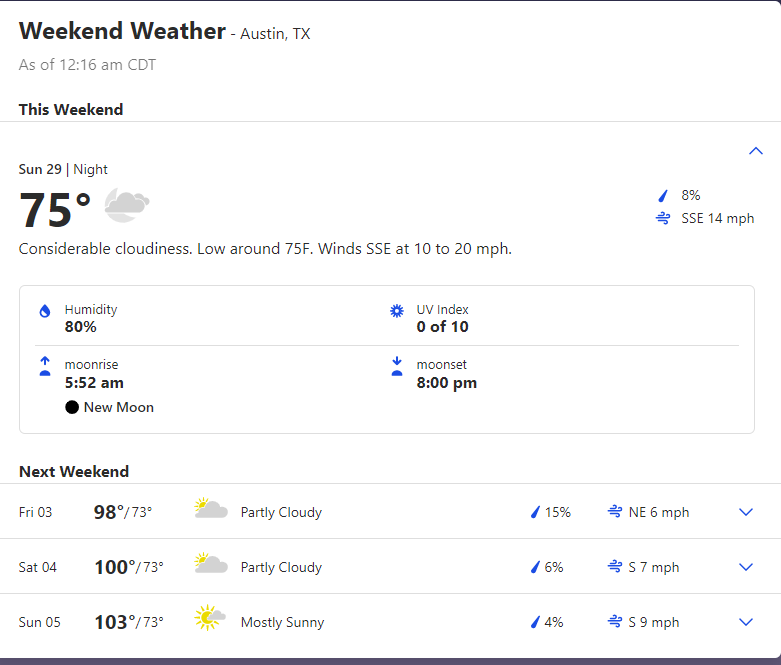The image is a screenshot from a device, likely a tablet or a larger phone, with a nearly square orientation displaying a weather forecast. The background is white with black or dark gray text. 

At the very top left, the header reads "Weekend Weather, Austin, Texas, as of 12:16 a.m. CDT." A section labeled "This Weekend" follows, with a dividing bar separating the details for "Sunday, 29th night, 75 degrees." An icon depicting a moon and clouds is positioned to the left and slightly above center. To the right of this icon, it states "8% SSE, 14 miles per hour."

Below these elements, a description reads, "Considerable cloudiness, low around 75°F, winds SSE at 10 to 20 mph."

In a gray box with a white background underneath, additional details include:
- Humidity: 80%
- UV index: 0 out of 10
- Moon rise: 5:52 a.m.
- Moon phase: New moon
- Moon set: 8:00 p.m.

Below this information, a list forecasts the weather for the next weekend, breaking down into:
- Friday: 98/73°F, partly cloudy
- Saturday: 103/73°F, partly cloudy
- Sunday: 103/73°F, mostly sunny

Icons representing clouds and the sun appear next to these temperatures. To the right are rain forecasts and wind details with drop-down options for further information.